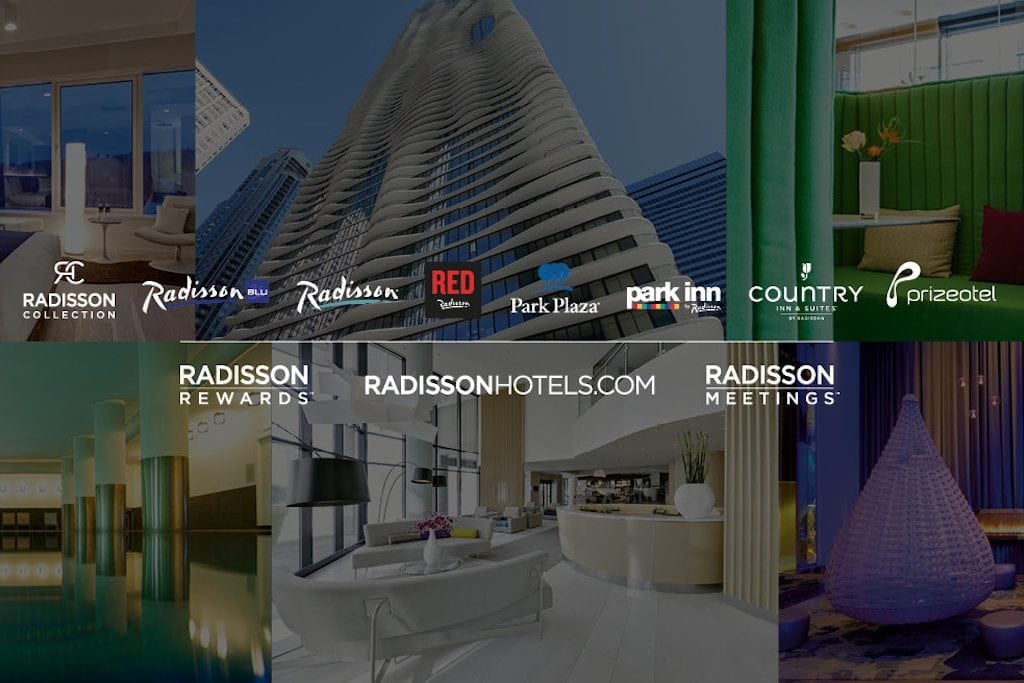A meticulously crafted graphic banner for Radisson showcases a collage of high-quality, professional photographs. At the center, a striking modern skyscraper dominates the downtown cityscape, its subtly twisting architecture with fin-like side details reaching toward the sky. Surrounding this focal point are grayed-out images displaying luxurious interiors: opulent rooms, elegant hallways, and grand ballrooms, each exuding sophistication and comfort. Superimposed on the collage are the names of various entities within the Radisson network including Radisson Collection, Radisson Blu, Radisson Red, Park Plaza, Park Inn, Country Inn & Suites, Prizeotel, Radisson Rewards, RadissonHotels.com, and Radisson Meetings. The entire composition not only highlights the extensive range and upscale nature of the Radisson brand but also conveys a sense of modern elegance and comprehensive hospitality services.